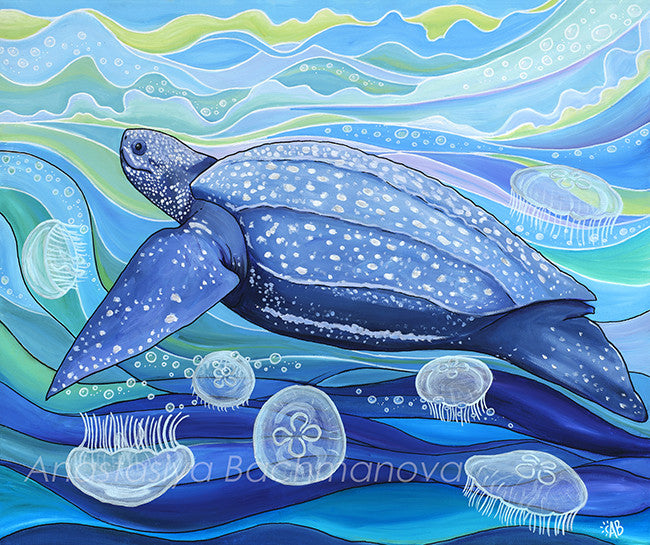The image is an artistic depiction of a turtle, most likely a sea turtle, painted in an abstract style. The turtle, centrally positioned and facing to the left, is rendered in various shades of blue and adorned with white spots that are smaller on its face and larger and more sparse on its back and fins. Surrounding the turtle are intricately detailed jellyfish, illustrated in different shapes and all painted in translucent white. The background is a mesmerizing blend of swirling colors, including blues, yellows, and light greens, with some swirls containing bubbles to enhance the underwater feel. Subtle white curvy lines traverse the image, adding to its dynamic and flowing nature. At the bottom, the name "Anastasia Bachmanova" is faintly inscribed in white font, indicating the artist, and there is a small signature "AB" with a half sun symbol in the bottom right corner.